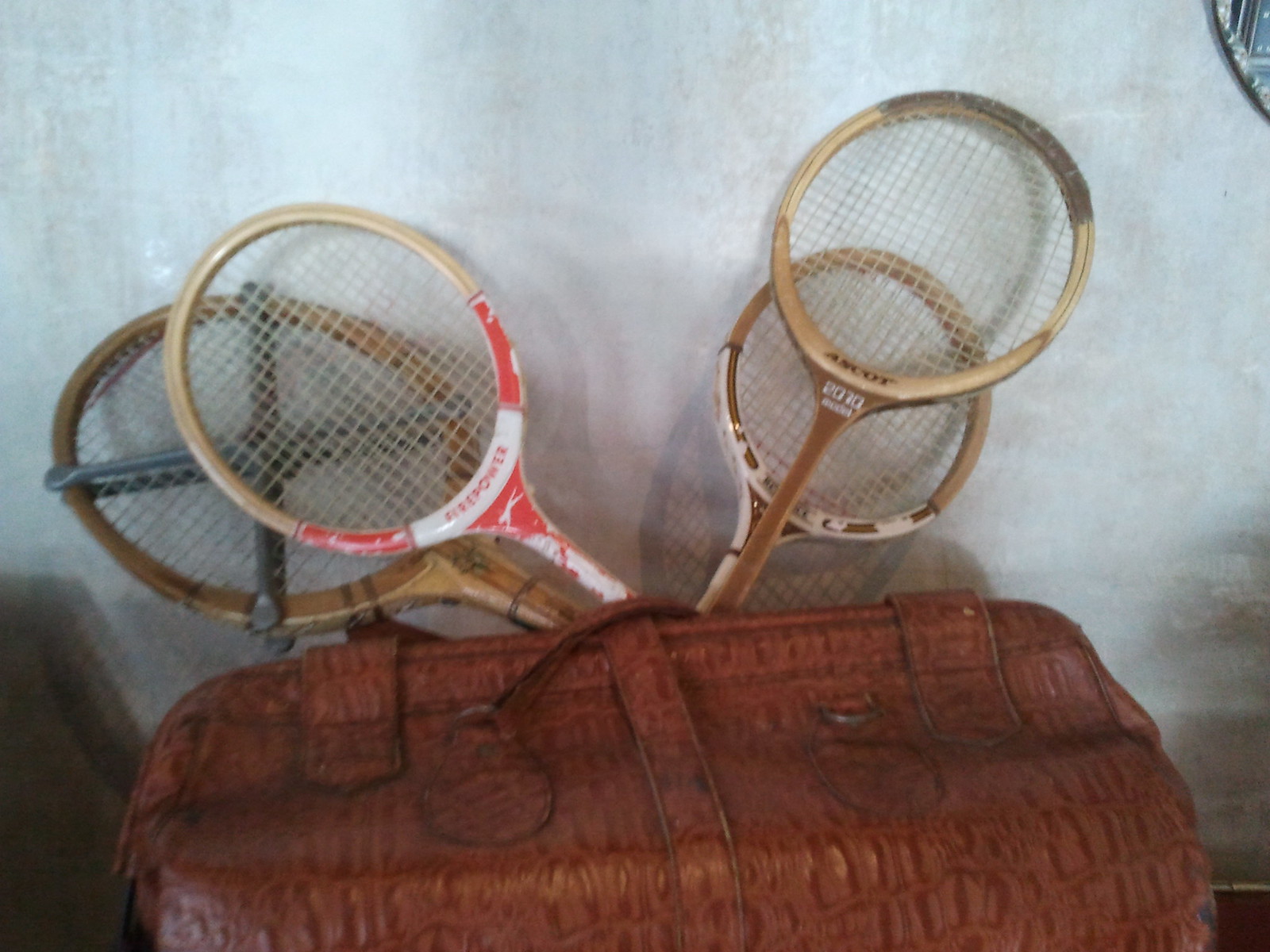This is an image of a reddish-brown leather bag, styled like a vintage carpet bag, with two clips to shut the top and a name tag hanging off it, though the name is not visible. Emerging from the open top of the bag are the handles of four vintage wooden tennis rackets. These rackets vary in appearance: one is a darker tan with black stripes and an X-shaped metal case around its strings; another is light tan with white and red stripes bearing unreadable wording; the third is light tan with black and white writing, including "Ascot"; and the fourth is light tan with worn-off paint showing hints of silver and gold. This assembly rests against a chalk-white wall, casting shadows due to direct light shining into the room.